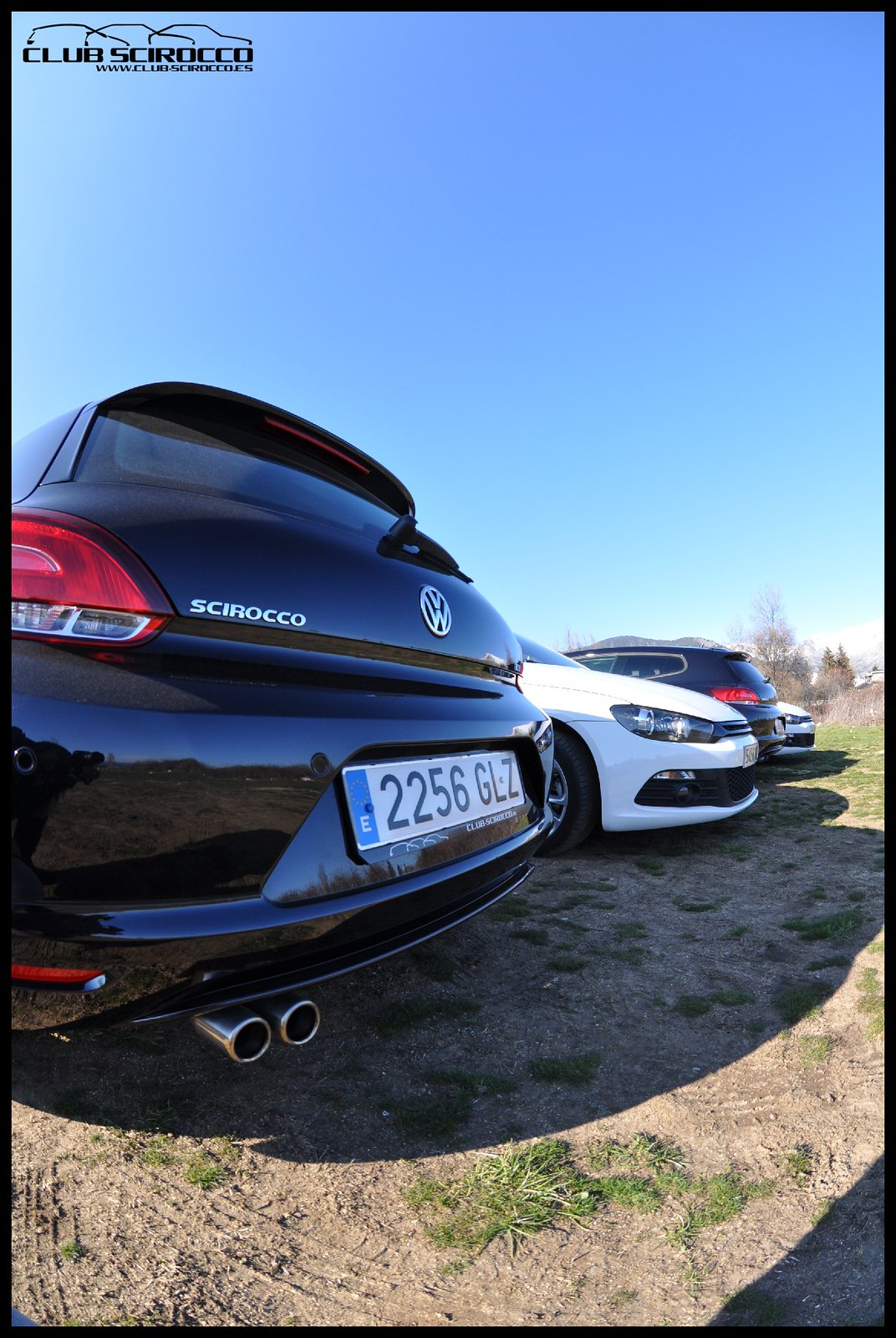This professionally shot photograph captures a lineup of four Volkswagen cars arranged in a grassy, dirt field under a bright, cloudless blue sky. Closest to the foreground, we see the rear of a dark blue-black VW Scirocco, prominently featuring a silver exhaust and a white license plate reading "2256 GLZ." Parked next to it, but facing the opposite direction, is a white sedan with its front end positioned where the Scirocco's rear is. Following the white sedan is a black SUV, parked with its rear in the same direction as the Scirocco. The sequence concludes with another white sedan, similarly reversed with its front pointing right. The background includes some trees, shrubberies, and distant mountains. In the upper left corner, the image bears the inscription "Club Scirocco," indicating a possible gathering or event for Scirocco enthusiasts.